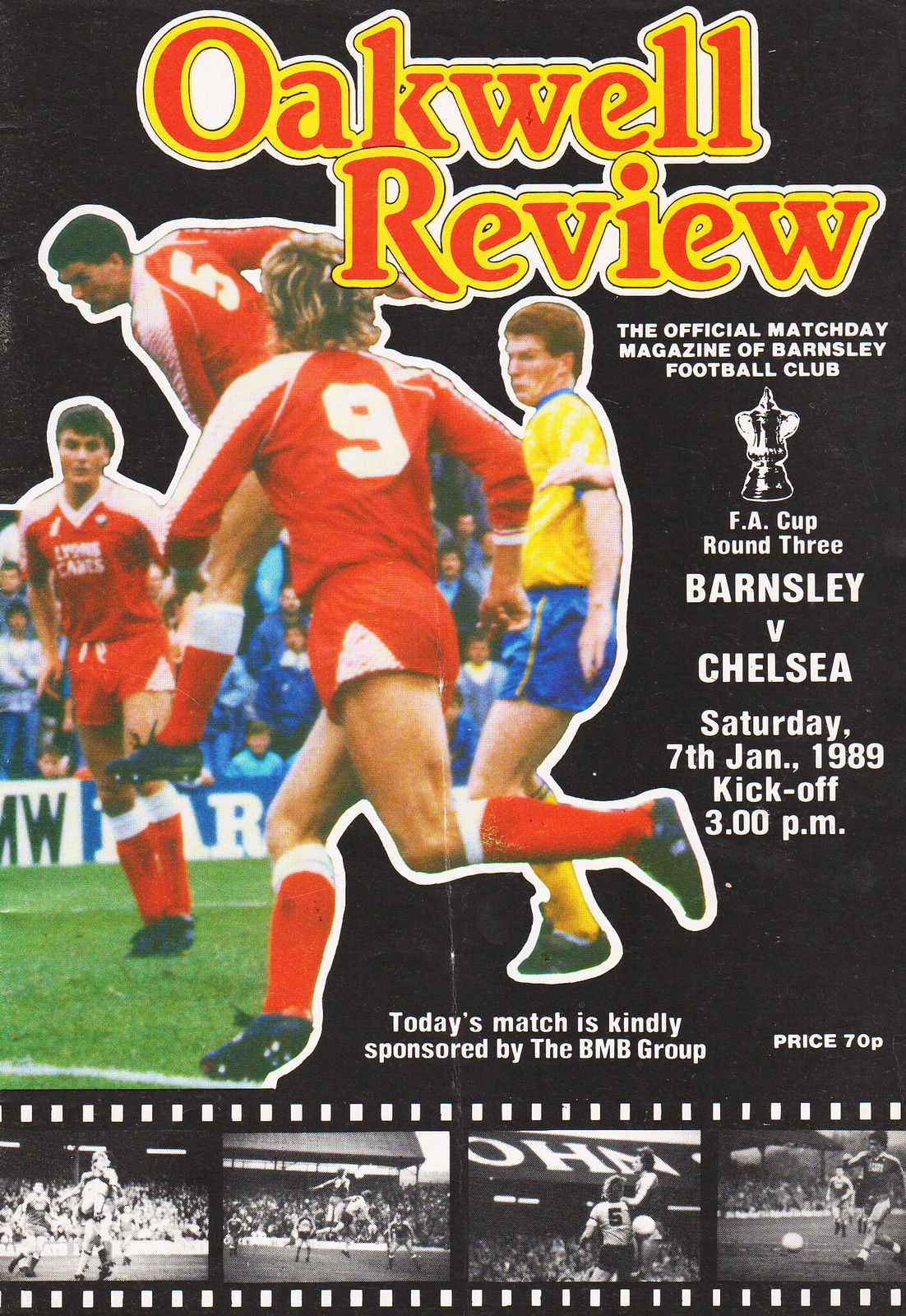The cover of the soccer match day magazine, "Oakwell Review," is vibrant and detailed. At the top, "Oakwell Review" is prominently featured in red letters outlined with yellow borders against a black background. Beneath this, in white font, it reads, "The official match day magazine of Barnsley Football Club." Next, the match details are provided: "FA Cup Round Three, Barnsley versus Chelsea, Saturday 7th January 1989, kickoff 3 p.m." A color photo of four players in action dominates the center; three players sport red jerseys, red socks, and black shoes, representing Barnsley, while an opponent in a yellow jersey with blue shorts is also visible. One Barnsley player appears to be in mid-air. The lower portion states, "Today's match is kindly sponsored by the BMB Group," and the program is priced at 70 pence. At the bottom, a film strip motif showcases black and white action shots of soccer gameplay, adding a dynamic and nostalgic touch to the magazine cover.